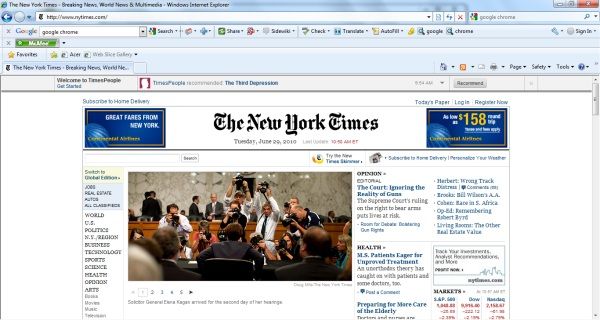In this image, we see a blurry screenshot of a web browser interface displaying the homepage of The New York Times. At the top, there is a white search bar set against a light blue background, with the URL "http://www.NewYorkTimes.com" displayed in bold black text above it. The title above the search bar reads "The New York Times - Breaking News, World News" and the browser is identified as Windows Internet Explorer. 

Beneath the search bar, there is a prominent Google logo, accompanied by another input bar with "Google Chrome" displayed to its right, followed by the word "Search". Despite the image's blurriness, the iconic New York Times masthead is discernable in bold black print. Adjacent to the title, on the left side, there is an advertisement promoting "Great Fares from New York" by Continental Airlines, presented in blue text. The lower portion of the screenshot is too blurry to make out any small text detail.